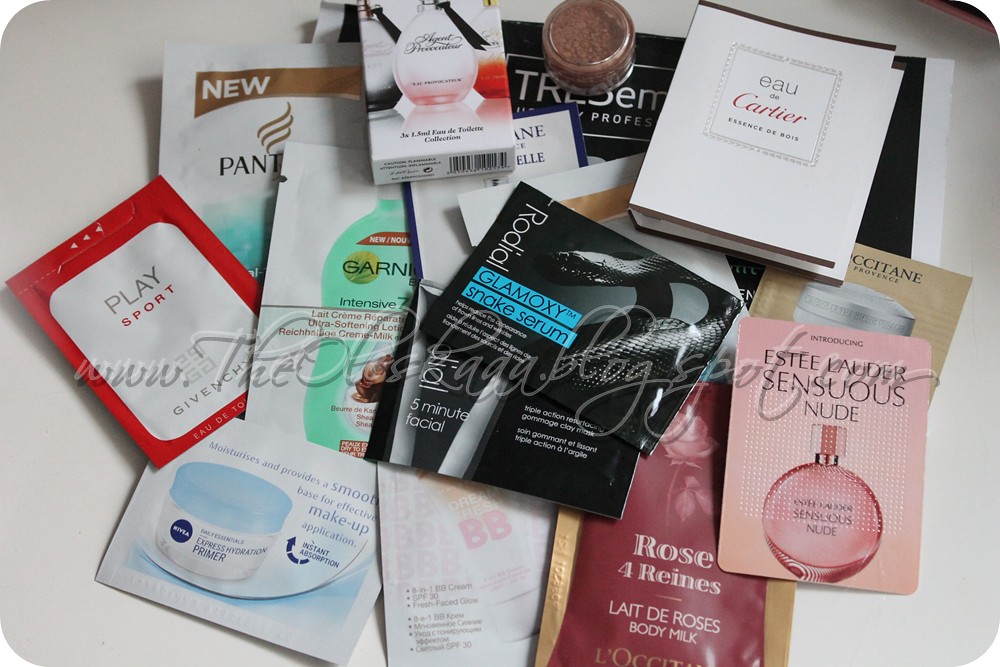This photograph showcases an array of beauty product samples meticulously arranged on a plain white background, with just the edge of a wooden table visible in the upper right corner, making it appear as though the products are on a slightly tilted whiteboard. The collection includes a small jar, several envelopes, a little box, and some pamphlet-like booklets, each partially overlapping the other. Featured items range from a sample of Givenchy's "Play Sport" to Nivea's "Instant Absorption" moisturizer. There is also "Rose for Greatness," a body milk labeled "Laid to Rose's," and a sample of "Sensuous Nude" by C.A. Lauder, which is likely a perfume. The arrangement suggests these are mostly sample products, offering a tantalizing glimpse into a variety of scents and skincare solutions.